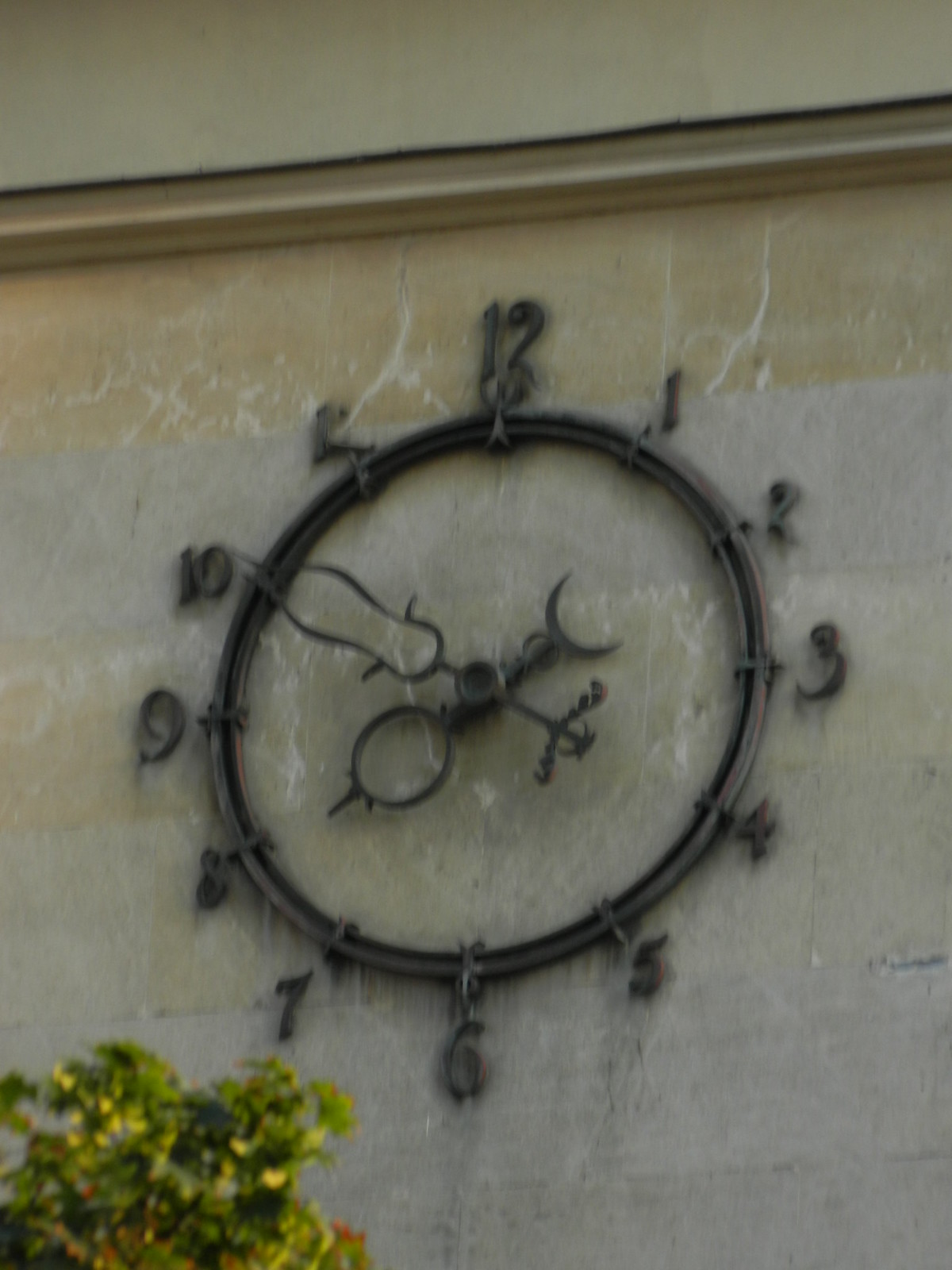This color photograph captures a unique and ornate clock affixed directly onto a dark gray stone wall made of light brown stone blocks arranged in subtle stripes. The clock, constructed from black iron or a similar metal, features a minimalist yet elegant circular metal ring with stylized numbers from 1 to 12 attached around its outer edge. The hands of the clock are particularly striking: the minute hand, resembling an item picker with a functional pointer, intersects with the center to form a stylized cross, while the hour hand is adorned with a sun motif on one side and a crescent moon on the other, with the sun pointing to the current hour. Positioned around the 7:50 mark, these hands add to the clock's distinctive design. At the bottom right of the image, a small, slightly blurred green plant, likely a bush or tree, adds a touch of natural color, complementing the textured stone background.